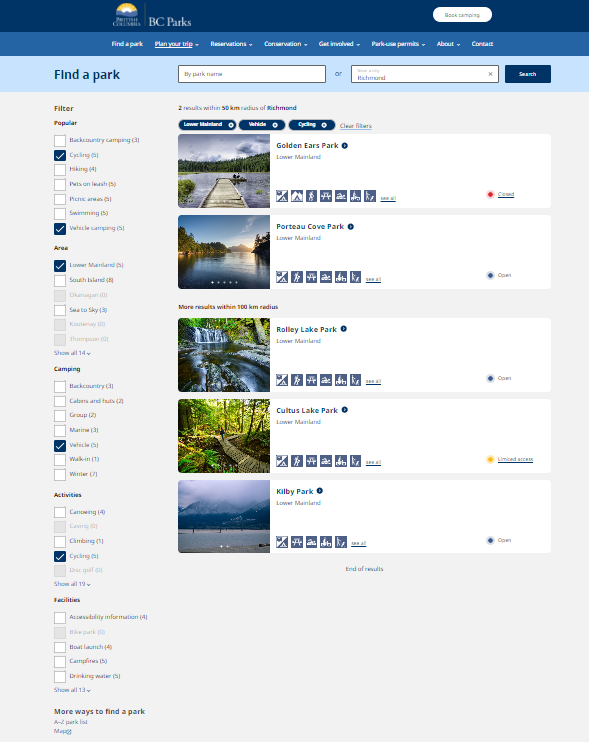This vertical image, likely from a website accessible via computer or smart device, displays a user interface for navigating the BC Parks website. At the top, a dark navy strip features "British Columbia" and an icon on the left, divided by a vertical line from the "BC Parks" text. To the right, a white button labeled "Book Camping" is visible. Below this, a lighter blue line contains clickable white text options: "Find a Park," "Plan Your Trip" (underlined), "Reservations," "Conservation," "Get Involved," "Park Use Permits," "About," and "Contact."

Further down, another lighter blue line highlights the "Find a Park" section. Here, users can search by park name or city, with a white search box displaying "Richmond" and a search button. To the left, filter options on a gray background allow selections by criteria such as cycling area, lower mainland, camping, and vehicle activities, with "cycling" currently selected.

In the middle section, highlighted results within a 50-kilometer radius of Richmond are shown. Each result includes an image, the park name, location details, various clickable icons, and indicators of whether the park is open or closed.